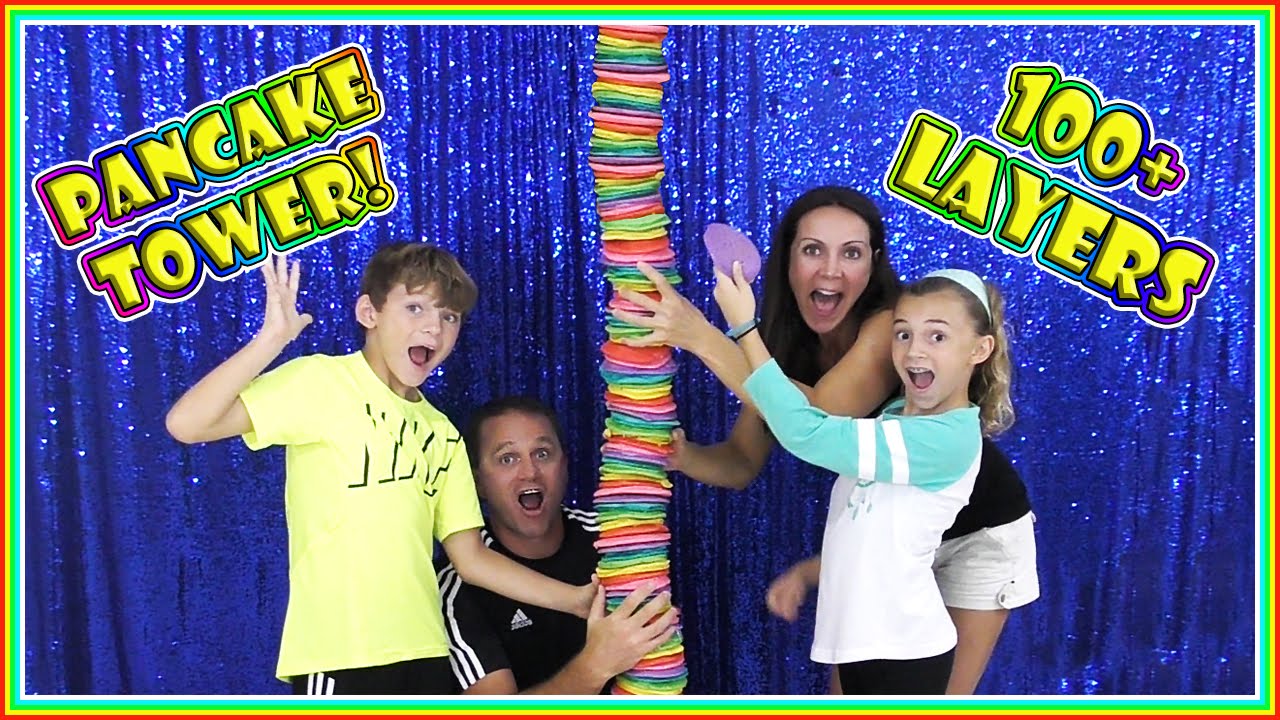The picture features a family of four, consisting of an older male, an older female, a young boy, and a young girl, all around 8 to 10 years old. They are posing with wide, open-mouthed expressions of surprise in front of a shiny, sparkly blue curtain backdrop, resembling streamers. The image is surrounded by multiple borders: a red border, followed by yellow, green, darker green, and finally white. At the top left, the words "Pancake Tower" appear in yellow with a rainbow border, while the top right has "100+ layers" written at an angle, also with a rainbow border.

In the center of the image stands an impressively tall, multicolored pancake tower featuring an array of vibrant hues such as green, pink, red, blue, yellow, and purple. The man, wearing a black Adidas shirt, is kneeling and holding the base of the tower. To his left, the boy with brown hair is dressed in a yellow Nike shirt, holding onto the tower with one hand and waving with the other. On the right side, the girl is gripping a purple pancake as if adding it to the tower, while the woman behind her, clad in a black shirt over a white one, helps to support the stack. All family members are looking at the camera, exuding excitement from their collective activity.